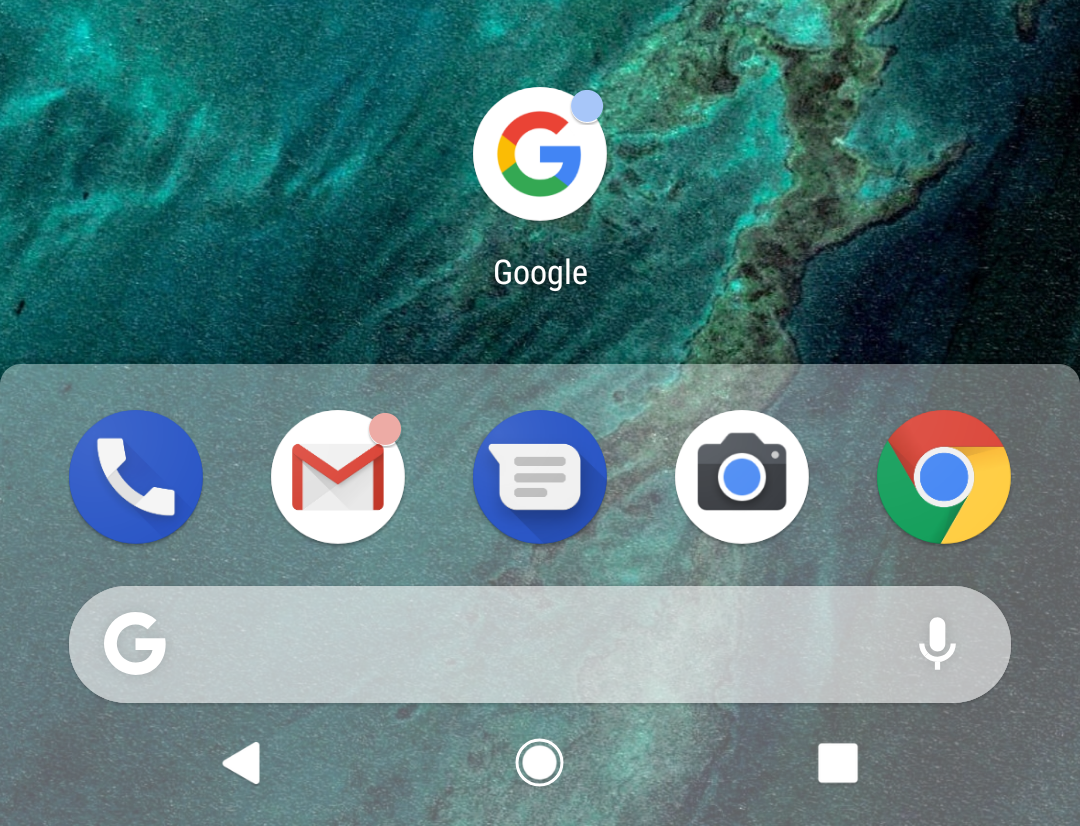The image depicts a screenshot of a Google search interface on a smartphone. The background features a vibrant topographic map showcasing diverse landscapes and water bodies. The hues range from various shades of green indicating land, to blue representing water bodies, with mountain ranges distinguishably marked in darker brownish-green tones.

Centrally positioned on the screen is the Google icon, a white circle containing the multi-colored "G" logo in red, yellow, green, and blue, with "Google" elegantly written beneath it. This central section is slightly muted by a shaded overlay, subtly blending with the colorful background.

Beneath the Google icon and text, a set of application icons is displayed. These include a blue circular icon featuring a white telephone symbol, indicating the phone app; the Gmail icon represented by an envelope with a bold, red "M"; a blue icon housing a white speech bubble for the messaging app; a white circular camera icon; and lastly, the Google Chrome icon symbolizing the web browser.

Below these app icons is a white search bar labeled with a "G" and includes a microphone icon for voice search capabilities. At the very bottom of the screen, navigation buttons are present: a left-pointing triangle for returning to the previous page, a circular home button at the center, and a square on the right for accessing recent apps.

This meticulously crafted interface highlights a seamless user experience, structured by clean lines and a balance of functional and aesthetic elements.